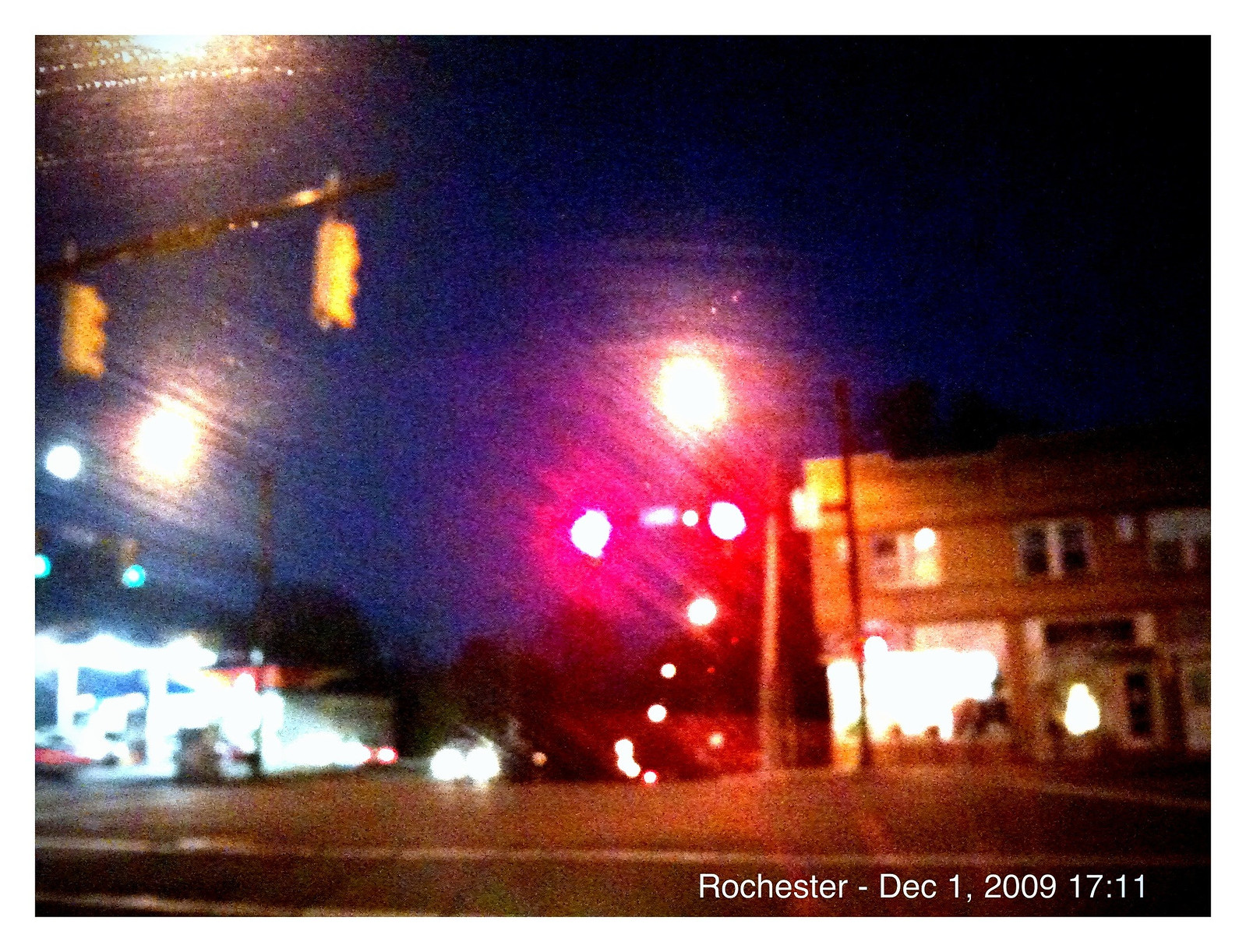This blurry, nighttime photograph, likely taken from a dash cam, is labeled at the bottom in white text: "Rochester - December 1, 2009, 17:11" (5:11 PM military time). The scene is set at an intersection in Rochester, either Minnesota or New York, as indicated. The sky is dark blue with the last remnants of sunset visible on the horizon. The intersection features a crosswalk at the bottom of the image, with traffic lights visible both facing the camera and facing away.

On the left side of the image, there is a gas station on the corner beneath green traffic lights for cross traffic. In front of the photographer, several cars' headlights shine, and a red light is visible in the center of the intersection. A fuzzy area around a large light in the center slightly obscures the view. To the right, there is a brown building with a glass-front, brightly lit for nighttime, alongside a tall pole. Silhouetted trees line the horizon in the background. Overall, the photograph captures a typical busy intersection with cars, buildings, and traffic lights under the darkening sky.